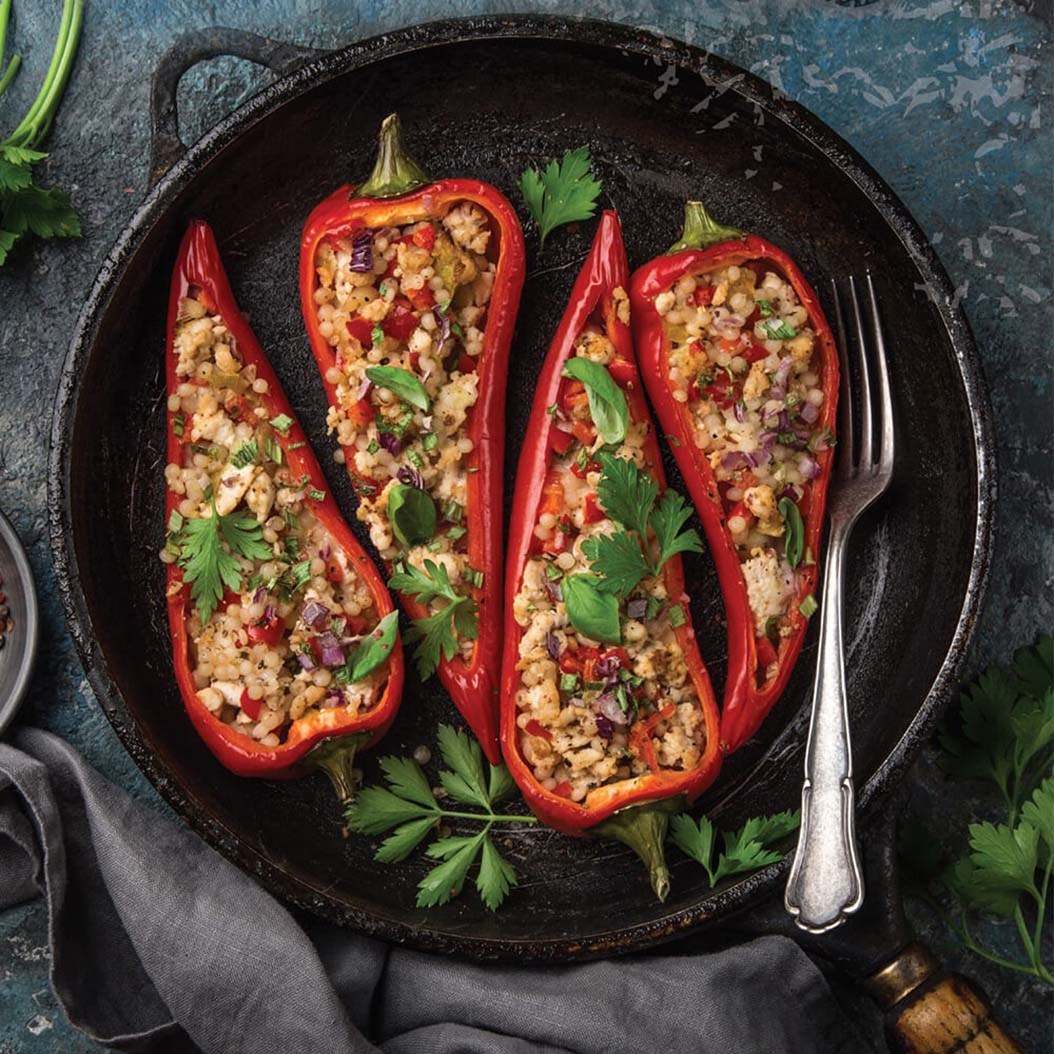An overhead, meticulously photographed shot showcases a black cast iron skillet with a wooden handle, resting on a dark teal stone table. The table is adorned with a dark gray napkin underneath the skillet and a silver fork positioned to the right. Inside the skillet, four halved, large red bell peppers stuffed with an inviting mixture of quinoa, purple onions, diced tomatoes, and green herbs, likely parsley, create a vibrant, rainbow-like appearance. The peppers are artfully arranged, highlighting chopped green herbs sprinkled both within and around them, enhancing the aesthetic appeal. This professional image, devoid of any text, exudes a high-end culinary excellence suitable for a gourmet magazine or cooking website.